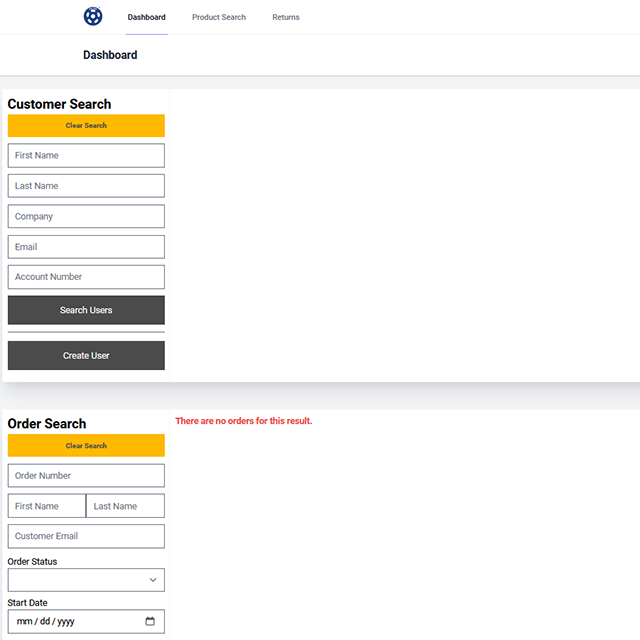In the app screenshot, the interface presents a clean and structured layout for user interaction. At the top left, there is a small logo featuring a blue star within a blue circle. To the right, three main navigation categories are displayed: "Dashboard" highlighted in black, "Product Search" in gray, and "Returns" also in gray.

The primary section below the navigation tabs is the "Dashboard" view. Spanning horizontally beneath this label is a light gray bar. The section immediately below includes a "Customer Search" feature, where a yellow search bar allows users to input search queries. User search criteria are divided into five fields: First Name, Last Name, Company, Email, and Account Number.

Towards the bottom of this customer section, two buttons are available: "Search Users" with a dark gray background and white text, and "Create User" with identical styling. The message "There are no orders for this result" is emphasized in red text, indicating a lack of results.

On the left side, there is an "Order Search" section with text in black. Right below, a "Clear Search" button is displayed in yellow. Search fields for orders include Order Number, First Name, Last Name, and Customer Email. Additional search parameters like "Order Status" and "Start Date" are also available for input.

The right-hand side of the interface features a predominantly white background interrupted only by another light gray horizontal bar, maintaining a consistent and minimalist aesthetic throughout the image.